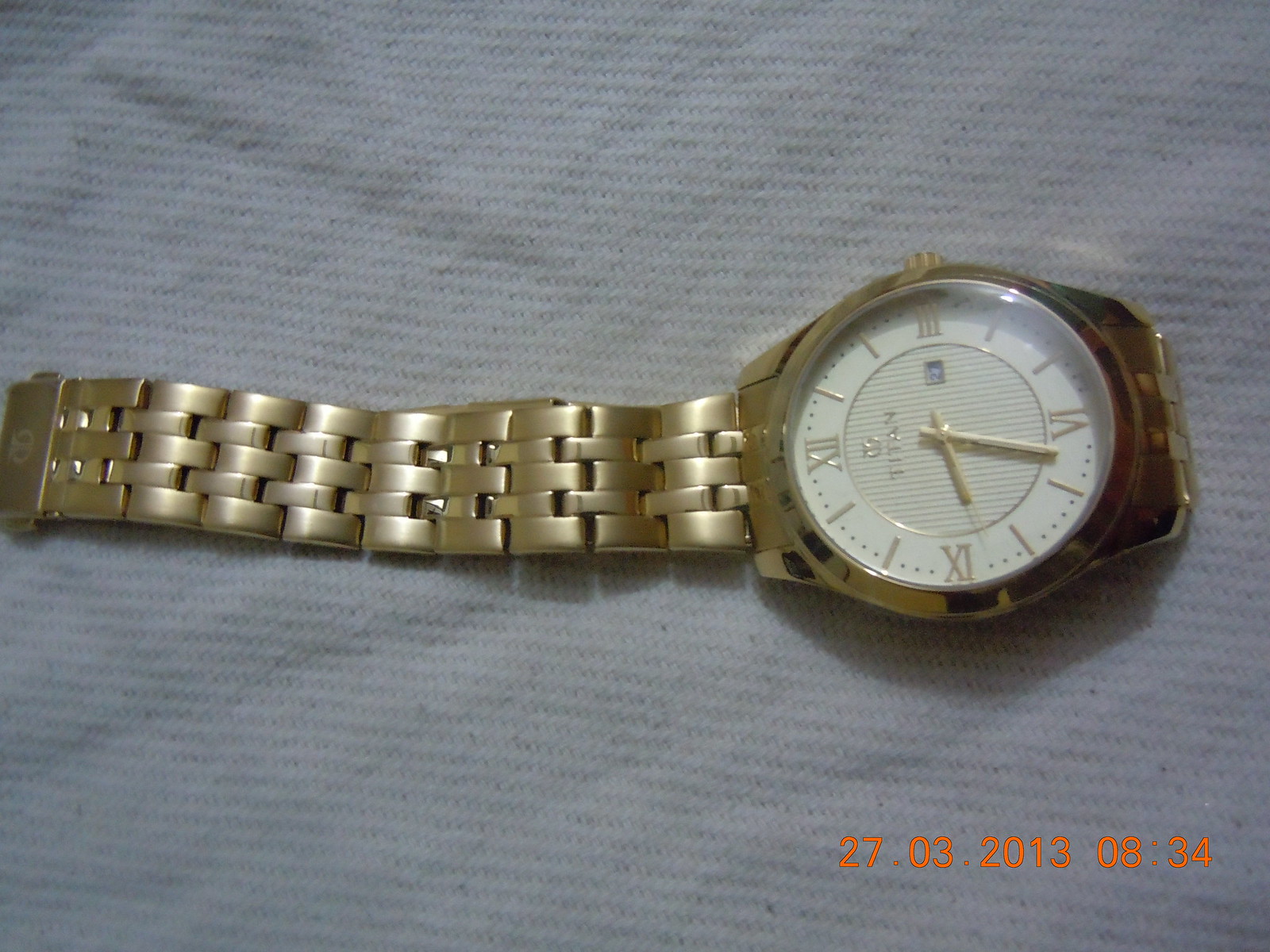This image features a meticulously detailed gold wristwatch resting atop a textured white fabric backdrop. The fabric, adorned with a subtle diamond weave pattern, contrasts elegantly with the opulent gold metal watch. The watch's band is composed of interlinked gold segments, creating a classic and luxurious appearance. Its face is a pristine white, elegantly complemented by gold Roman numerals indicating the hours. The watch's hour, minute, and slender second hands are also crafted from gold, harmoniously blending with the overall design. Inscribed in bold orange at the bottom of the image is the date and a series of numbers: "27.03.2013.0834," adding a unique timestamp to the composition.